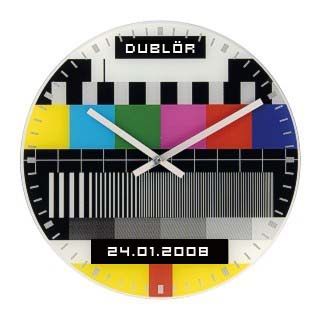Here we have a unique and artistic wall clock set against a plain white background, giving it a minimalist feel perfect for mounting. The design is reminiscent of a TV test pattern with vibrant colored squares in green, pink, red, navy blue, baby blue, and yellow, interspersed with black and white, echoing the familiar static screen from older television sets. Notably, the clock face lacks numerals, featuring only hash marks for a modern, 8-bit, computer-inspired aesthetic, almost like barcodes. The hands of the clock point to around 10:10, a time commonly used in advertisements. Intriguingly, the clock displays the date January 24, 2008, in the format 24.01.2008. At the top, it bears the inscription "Dublör," with an umlaut over the 'O', suggesting perhaps a German influence or origin.